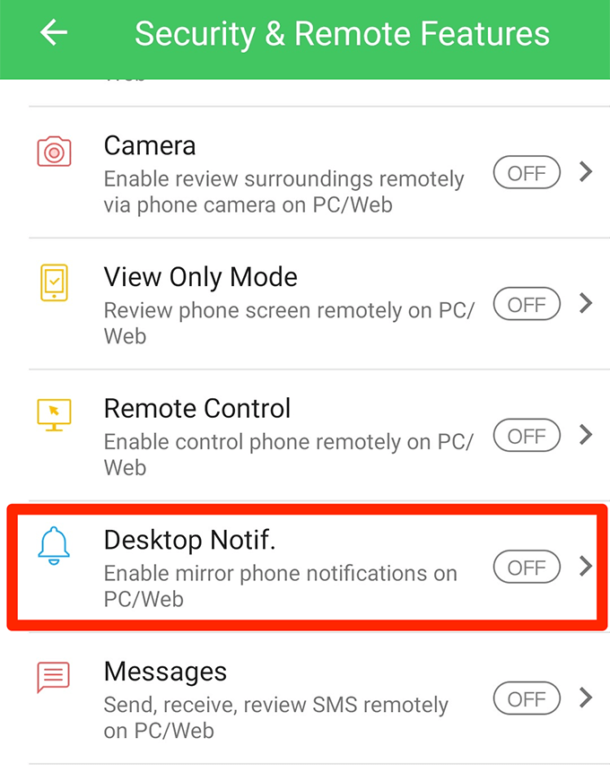The image is a screenshot from a smartphone displaying a security and remote features menu against a white background. At the top, there is a green banner with "Security and Remote Features" written in white font. In the upper left-hand corner, there is a white arrow pointing to the left.

Below the banner, the content is listed in black font. The first item is labeled "Camera" and is accompanied by a simple red drawing of a camera. It includes the description: "Enable review surroundings remotely via phone camera on PC/web."

Following that, the second item is "View Only Mode," which states: "Review phone screen remotely on PC/web."

The next item is "Remote Control," described as: "Enable control phone remotely on PC/web."

The final item is highlighted with a red-outlined rectangle. It is labeled "Desktop Notif" (abbreviation for Notification) and includes a blue bell icon, indicating notifications. The description reads: "Enable mirror phone notifications on PC/web."